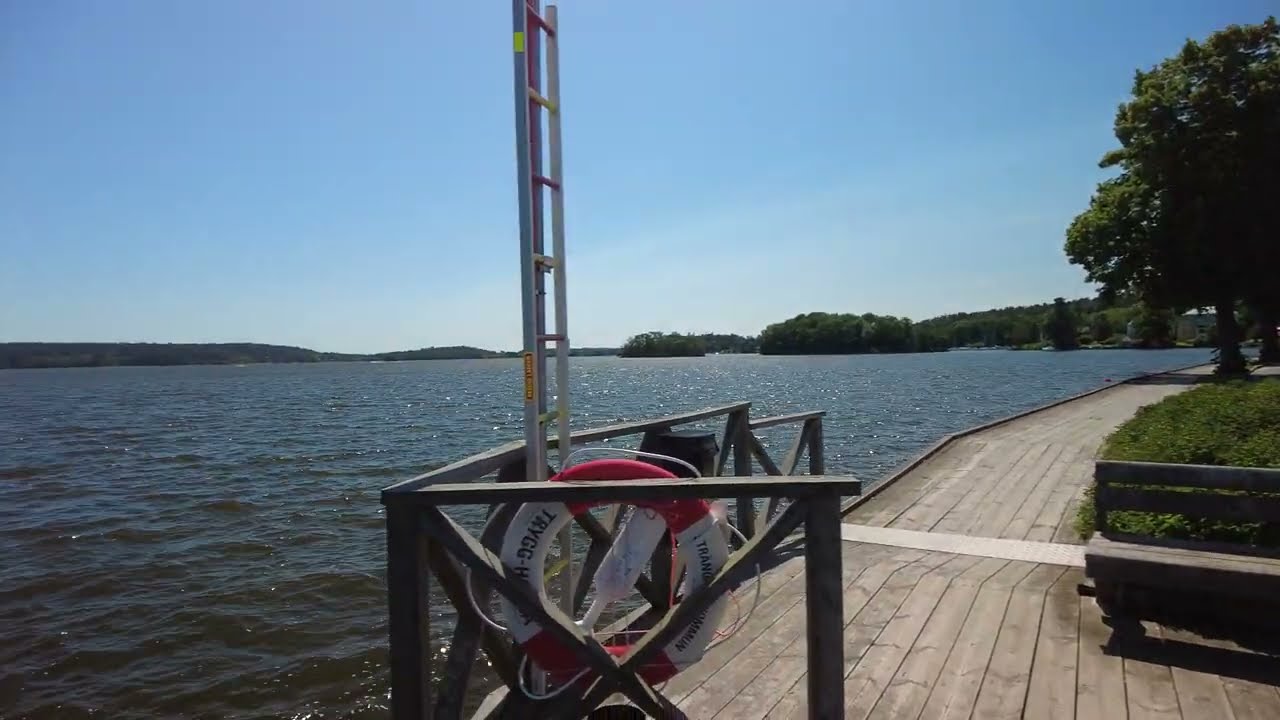In the bright, sunny image of a lakeside scene, a distinctive walking chair with vertical wooden panels stands prominently on the right side. Adjacent to it is a wooden bench, surrounded by lush vegetation and a tall, fluffy tree. The scene is framed by a wooden fence adorned with red and yellow sections, which guides the eye towards a central lifeguard station. This station features a straight vertical ladder leaning against a wooden railing, with a red and white lifesaving buoy attached. The murky yet serene lake waters stretch out from the left, exhibiting slight choppiness with white caps, and extend to the far background where verdant low mountains filled with green plants rise beneath the clear, vibrant blue sky.